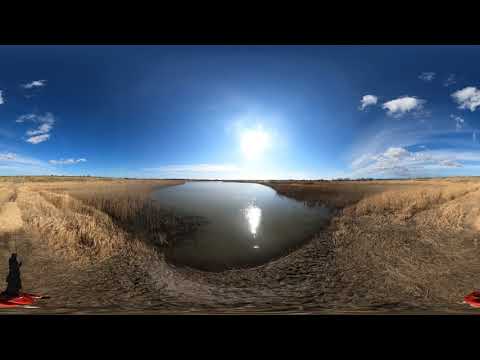The image depicts a 360-degree panoramic view of an outdoor scene dominated by a tranquil, marshy lake. The lake, which shows a dark gray and somewhat muddy appearance, is surrounded by dry, light tan, and brown reeds, creating a stark contrast with the clear blue sky overhead that features a scattering of white clouds. The bright sun, centrally located in the sky, casts a glaring reflection on the calm surface of the water. Extending from the foreground across the panoramic scene, patches of dead, dry grass frame the lake on both sides. There is a dirt path leading to the water's edge, hinting at potential human activity. In the lower left corner of the image, a red object, possibly a chair or part of some outdoor equipment, is visible, with a silhouette or shadow near it suggesting the presence of a person, potentially fishing. The distinct black borders at the top and bottom of the image emphasize its fish-eye effect, giving it a unique and immersive perspective.